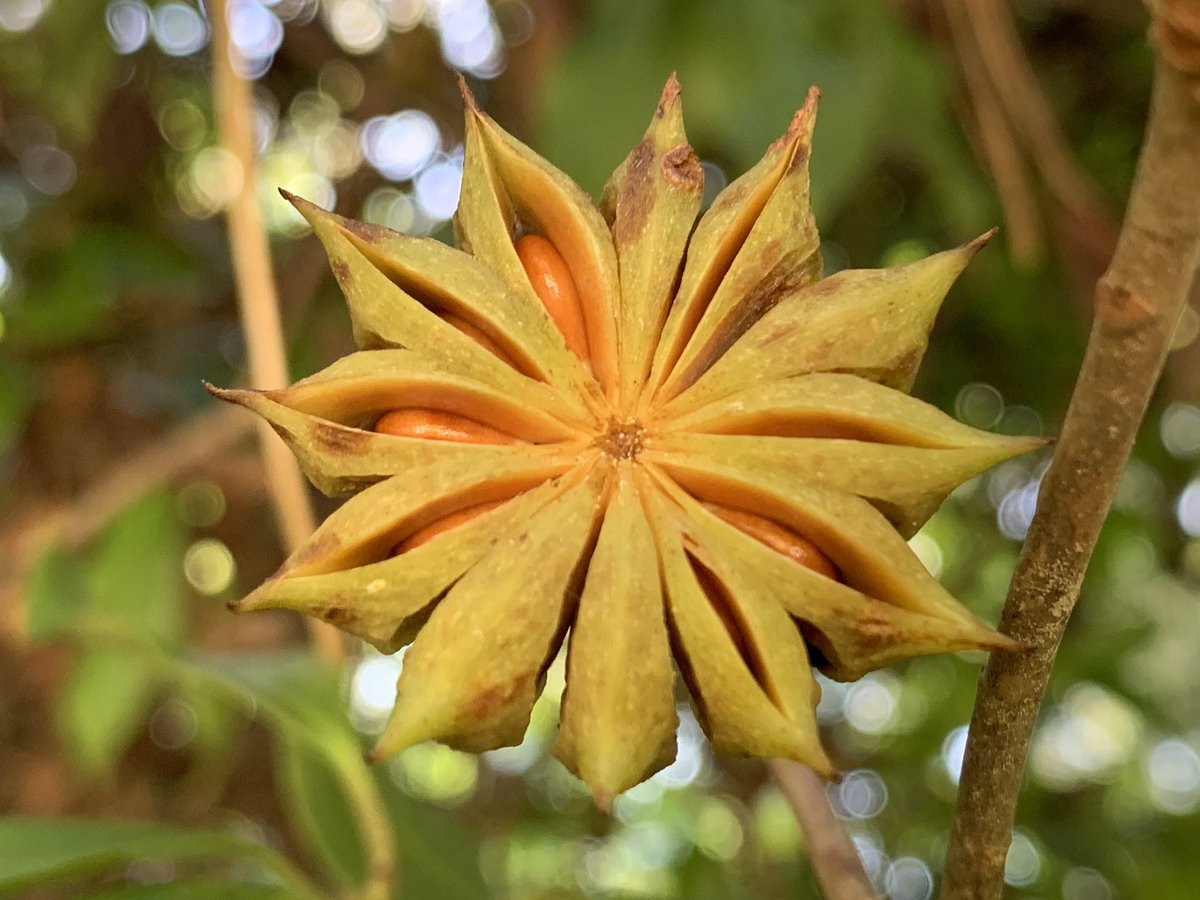This close-up photograph captures a unique star-shaped fruit with approximately 10 to 12 arms. The fruit is a captivating mix of green and yellow on the outside and contains an orange, edible substance in the slits between its arms. The texture of the fruit's exterior resembles that of a melon or pineapple, with a somewhat creamy or rubbery appearance. Attached to a small brown branch, the fruit is still connected to the tree. In the blurred background, hints of green and brown represent leaves and branches of surrounding trees, with small blue dots suggesting the sky.